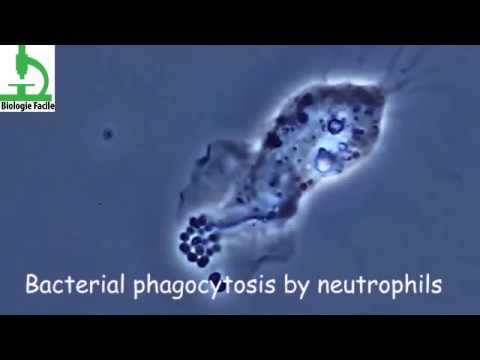This image, likely taken from a microscope, prominently displays bacterial phagocytosis by neutrophils. The background is predominantly blue, with a large, diagonally oriented bacterial cell also stained blue at the center. The image is bordered by black at the top and bottom, where white text clearly labels the process: "bacterial phagocytosis by neutrophils." In the top left corner, there is a distinctive green illustration of a microscope with the phrase “biology fowl” written below it in black text.